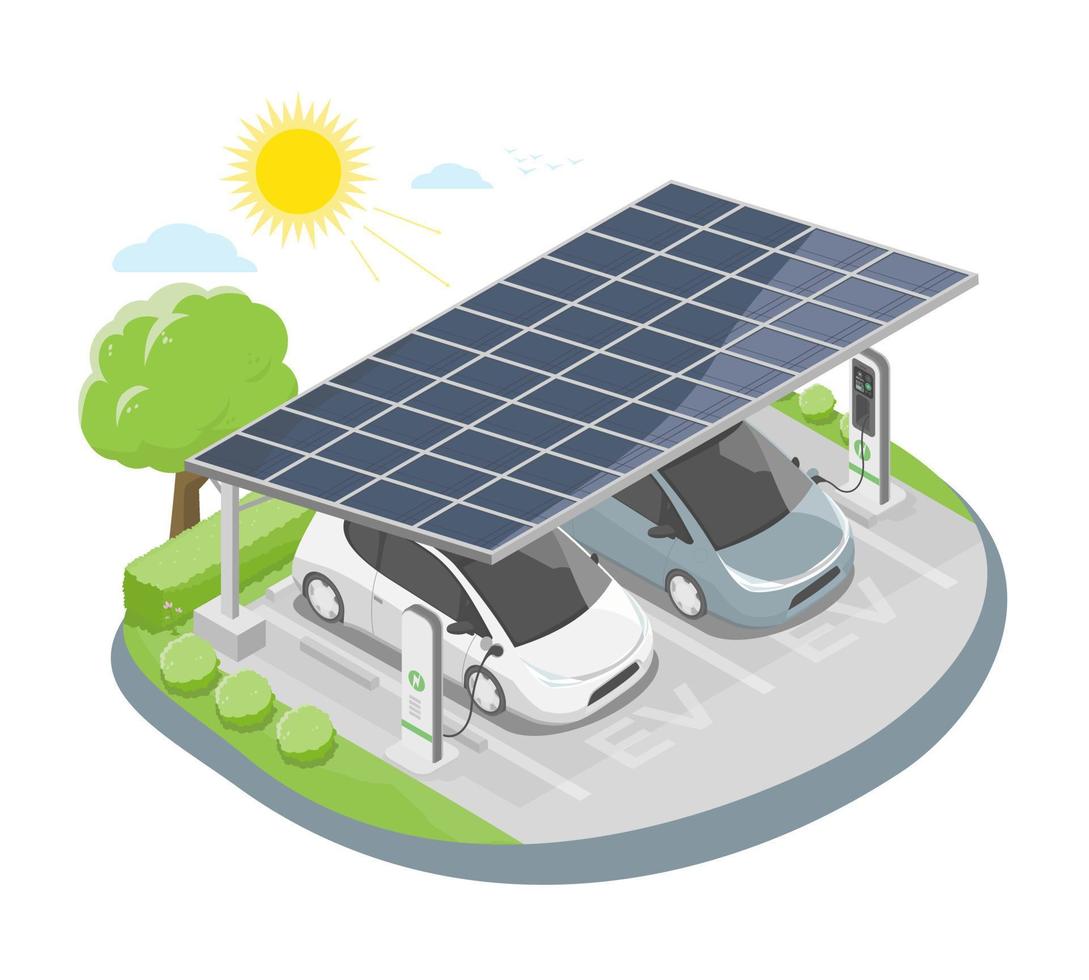The image is a detailed drawing representing the solar-powered charging of electric vehicles, depicted in a cartoon style. The focal point is a large, dark blue solar panel that forms an awning over two parked cars—a white one and a light blue one. These cars are connected to nearby charging stations. The ground, a light gray surface, has the letters "EV" written in front of each parking space. Surrounding this setup, there is a simple landscape featuring green bushes on both sides and behind the charging area, along with a prominent green tree directly behind the cars. The sky above is adorned with a bright yellow sun, some blue clouds, and a couple of birds, while the rest of the background remains white. The overall sketch clearly highlights the eco-friendly approach of using solar energy for charging electric vehicles.